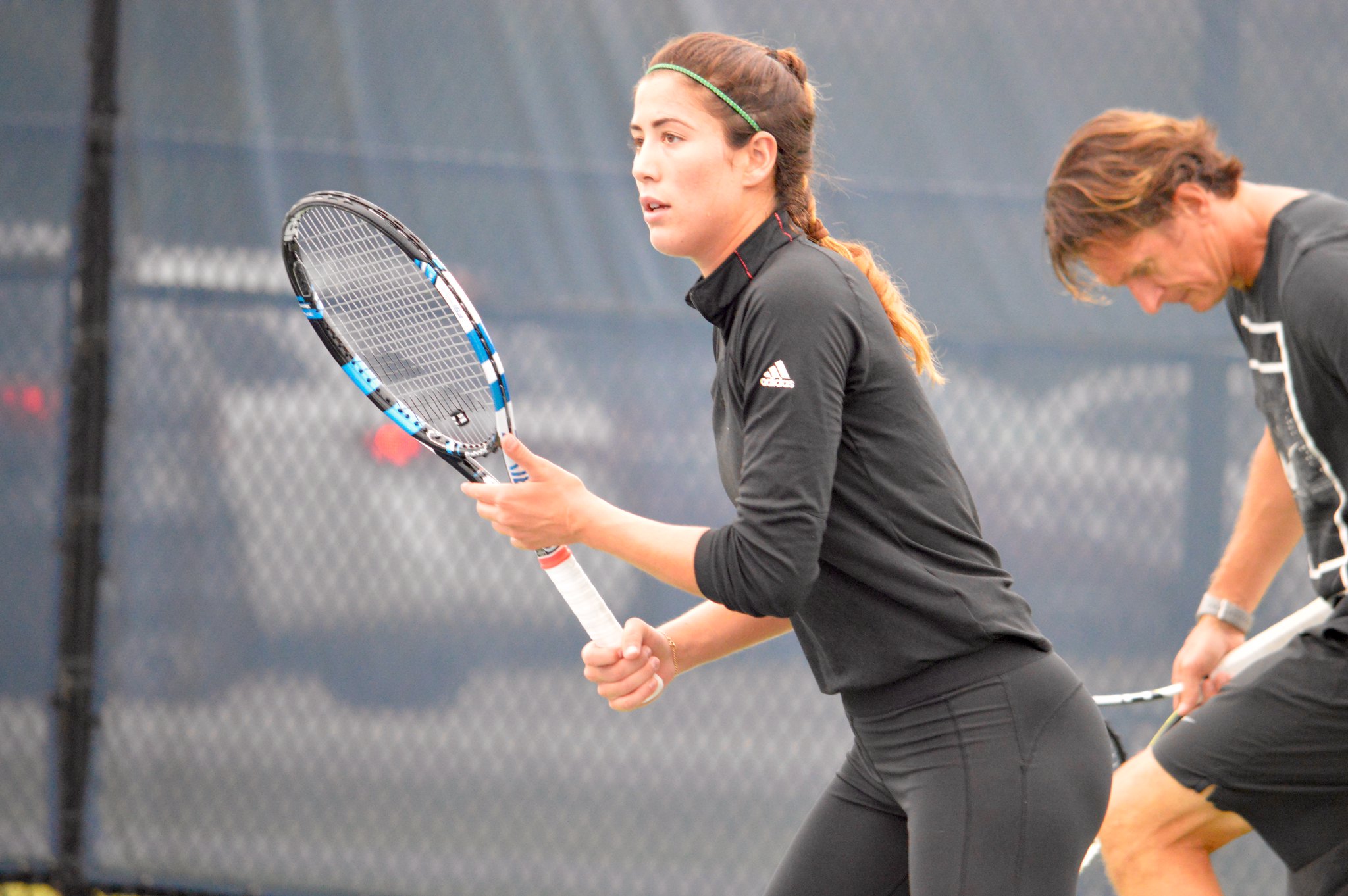In this dynamic tennis court scene, two players are captured in action against the backdrop of a woven chain-link fence. The young woman, poised to make a decisive move, stands with her racket raised, ready to strike an incoming ball. She sports sleek black Adidas leggings and a tight jacket bearing the brand's logo. Her reddish-brown hair, intricately braided, falls gracefully to the middle of her back, complemented by a thin green striped headband. Just behind her to the right, a man in a casual gray t-shirt adorned with a graphic on the front and black shorts intently observes the game. His wristwatch catches the light as he holds his racket in his right hand, somewhat obscured by the girl's stance. His mid-length hair frames his face as he focuses on the unfolding match, adding to the anticipation and intensity of the moment.